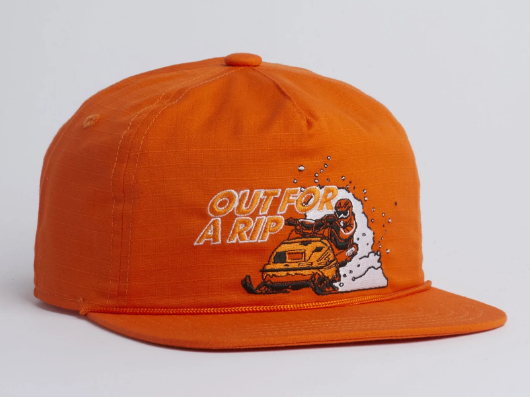The image is a rectangular, commercially-styled photograph of an orange baseball cap set against a continuous white background. The cap has a flat brim and features a button on the top. It is meticulously stitched with lighter orange threads, adding to its detailed construction. Centered on the front panel, in orange embroidery bordered with a thin white outline to make it pop, are the words "Out for a Rip." Below the text, there is a cartoon-style depiction of a person in an orange suit riding an orange snowmobile, leaving a trail through a patch of snow. This image is geared towards an online commercial setting, focusing attention solely on the product.